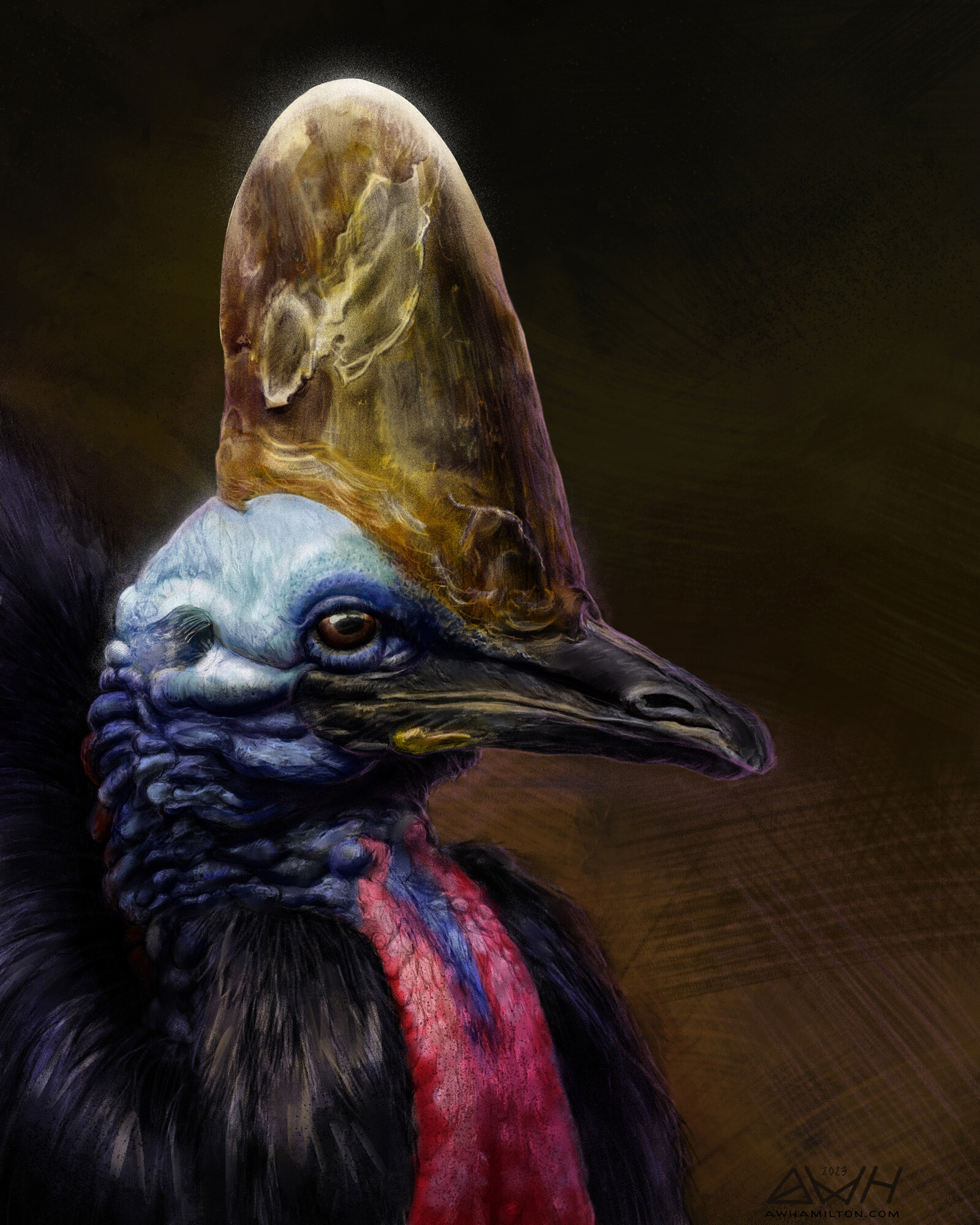This is an artistic painting of a unique bird set against a brown, pencil-marked background with a plaid-like texture. The bird, which dominates the composition by soaring from the bottom left to the center and top of the canvas, is strikingly detailed. The bird's body is dark brown, adorned with a vertical red stripe down its chest resembling a tie, and a smaller blue stripe above it. Its neck is textured with small, corn-like pieces, transitioning from blue at the top to a red, wattle-like skin beneath. The bird's head is light blue, gradually darkening around the eyes, which are brown with black centers. Its black beak features a gold mouth line. Situated above its head is a large, helmet-like protrusion in a swirled pattern of tan and brown, almost reminiscent of a half-moon shape. The bottom right-hand corner of the painting features the website address "AWHAMILTON.com" alongside a triangle logo representing an A, W, and H, dated 2019.